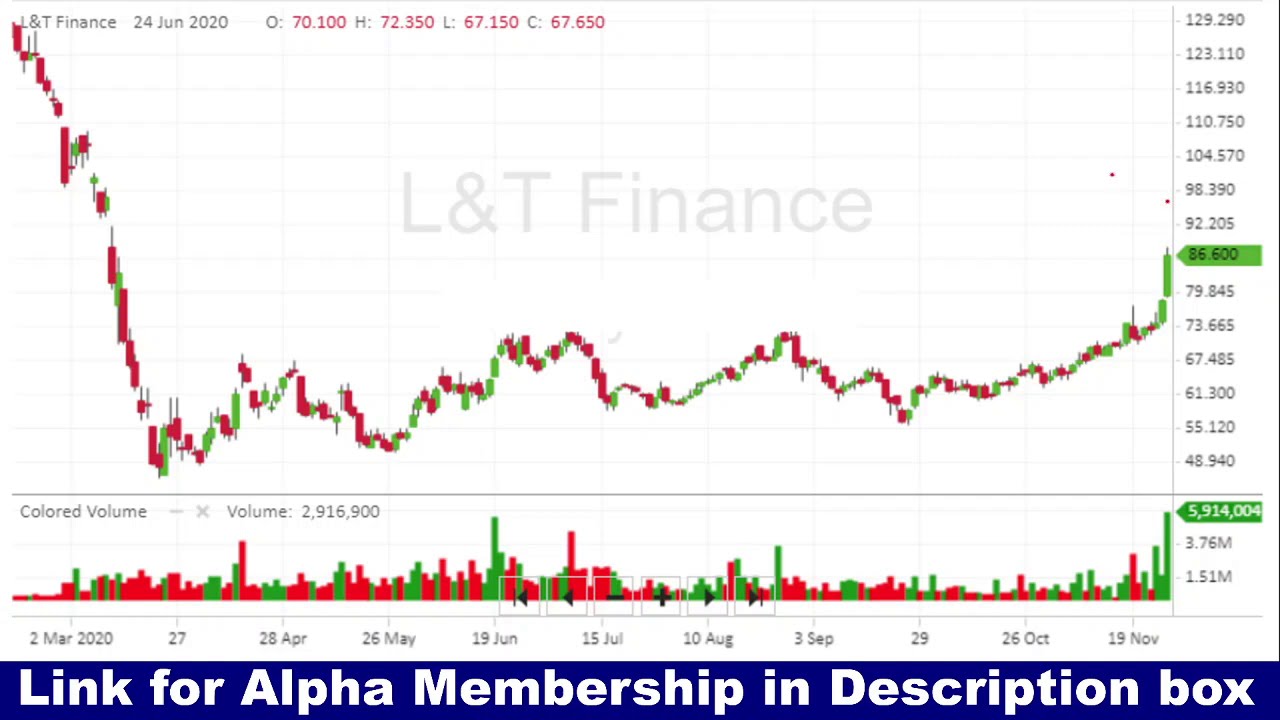The image is a screenshot from a finance video, depicting a detailed candlestick graph of L&T Finance. At the top left, the graph is labeled with small text reading "L&T Finance" and dated June 24, 2020. The backdrop is white, and the graph showcases the movement of L&T Finance stock, with red and green candlesticks representing day-to-day price fluctuations. These candles illustrate the highs and lows of the stock, starting from March 2, 2020, with notable sharp dips and subsequent fluctuations. On the right side of the graph are numerical values ranging from 129.290 down to 48.940. Along the bottom, it is noted that the stock volume is 2,916,900, and the dates range from March 2, 2020, to November 19, 2020. A blue banner at the bottom of the image provides additional information, stating "Link for Alpha Membership in description box." The grid of the graph also features a watermark that reads "L&T Finance."